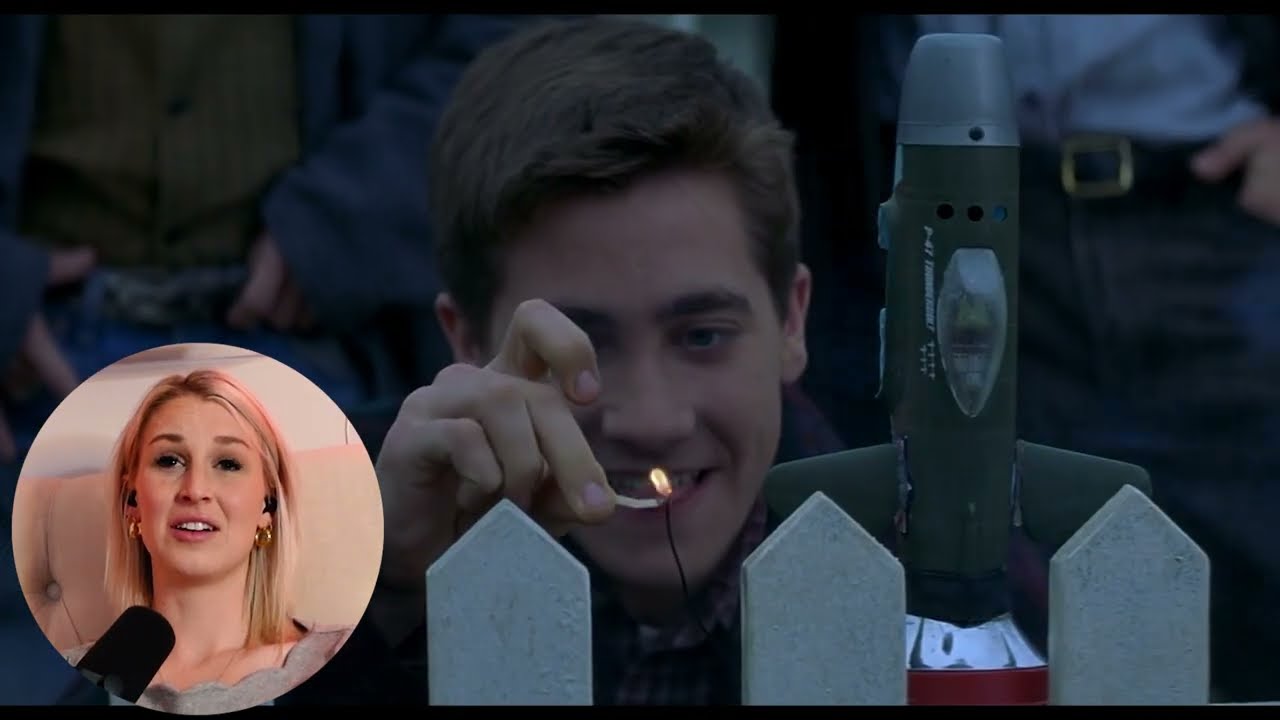In this image, the central focus is a young boy with brown hair and white skin, intensely concentrating as he uses a match to light the fuse of a green rocket. This rocket, which has a silver top and a red tail, stands slightly to the right of the boy, who is directly in the center of the image. A couple of observers, visible from the waist down, are standing behind him, also seeming to watch the event. This scene is partly obscured by a light black overlay but remains discernible.

In the bottom left corner of the image, there is a circular inset showing a detailed and in-focus view of a woman who appears to be reacting to the boy lighting the rocket. She has long, flowing blonde hair, and her face is framed by two sets of gold earrings. She wears a gray top with an open neckline and sits comfortably on a tan couch with a white wall behind her. The woman is speaking into a black microphone and her expression is one of engrossed attention.

The overall setting suggests an outdoor celebration, perhaps a scene from a movie, which the woman is likely reacting to as a content creator. The image does not contain any text, and the predominant colors are tan, white, yellow, black, gray, red, and blue. The picture captures a vivid moment of anticipation and reaction, seemingly blending a personal live commentary with an engaging visual narrative.